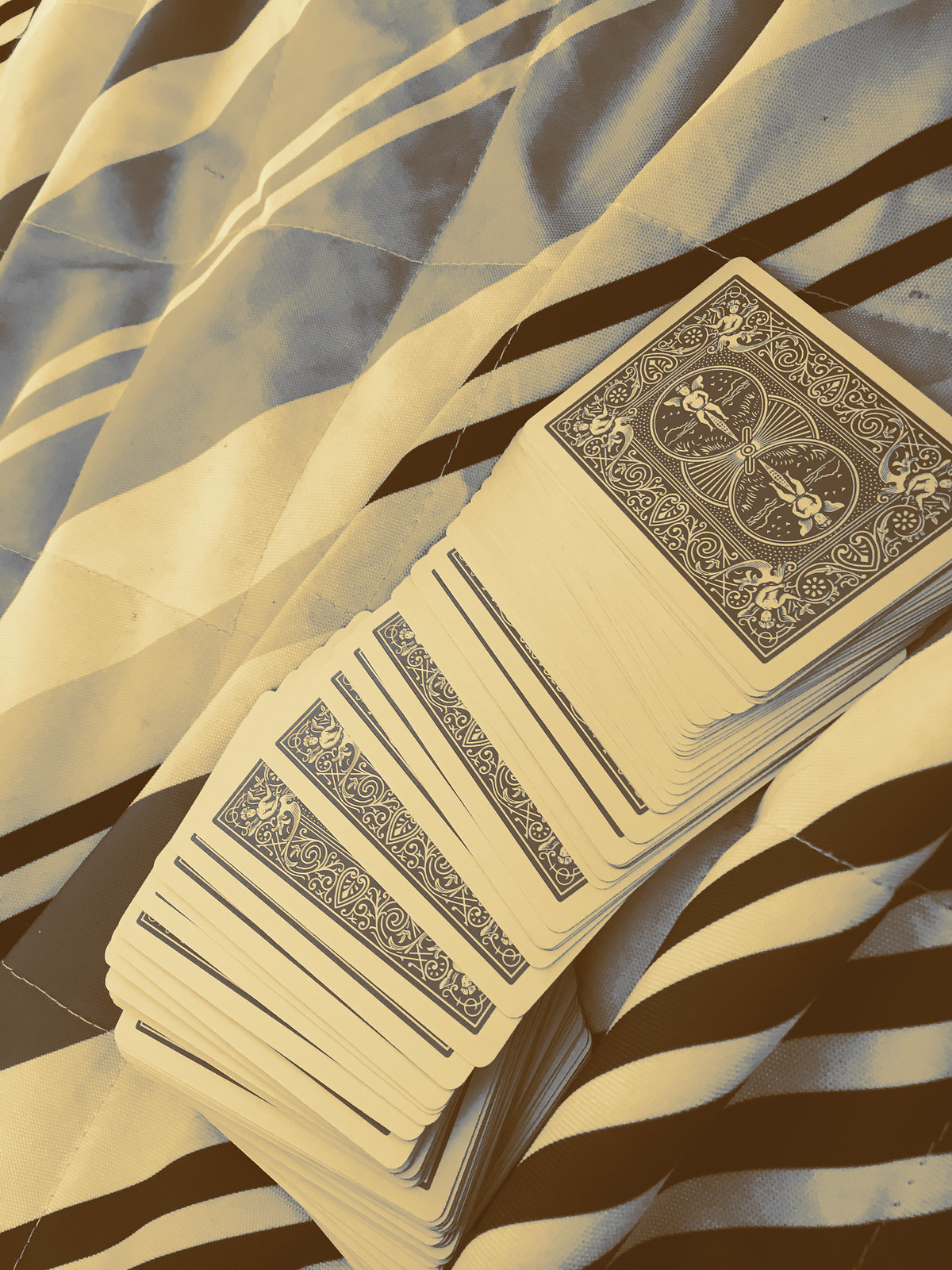A deck of cards is spread out gracefully atop a white cloth adorned with brown and gray stripes, giving the scene a sophisticated yet cozy ambiance. The photograph captures a warm, brownish tint, adding a vintage feel to the setting. The back of the cards features an elaborate gray and white design, highlighting three interconnected circles at the center. A character appears to be standing within two of these circles, while the central circle is embellished with fine lines. The elaborate border showcases a pattern reminiscent of waves, with representations of sea creatures in each corner. Their long tails curl elegantly around the edges, integrating with the intricate swirls that frame the cards. The cloth underneath, displaying visible stitching and light reflections, adds texture and depth to the composition.